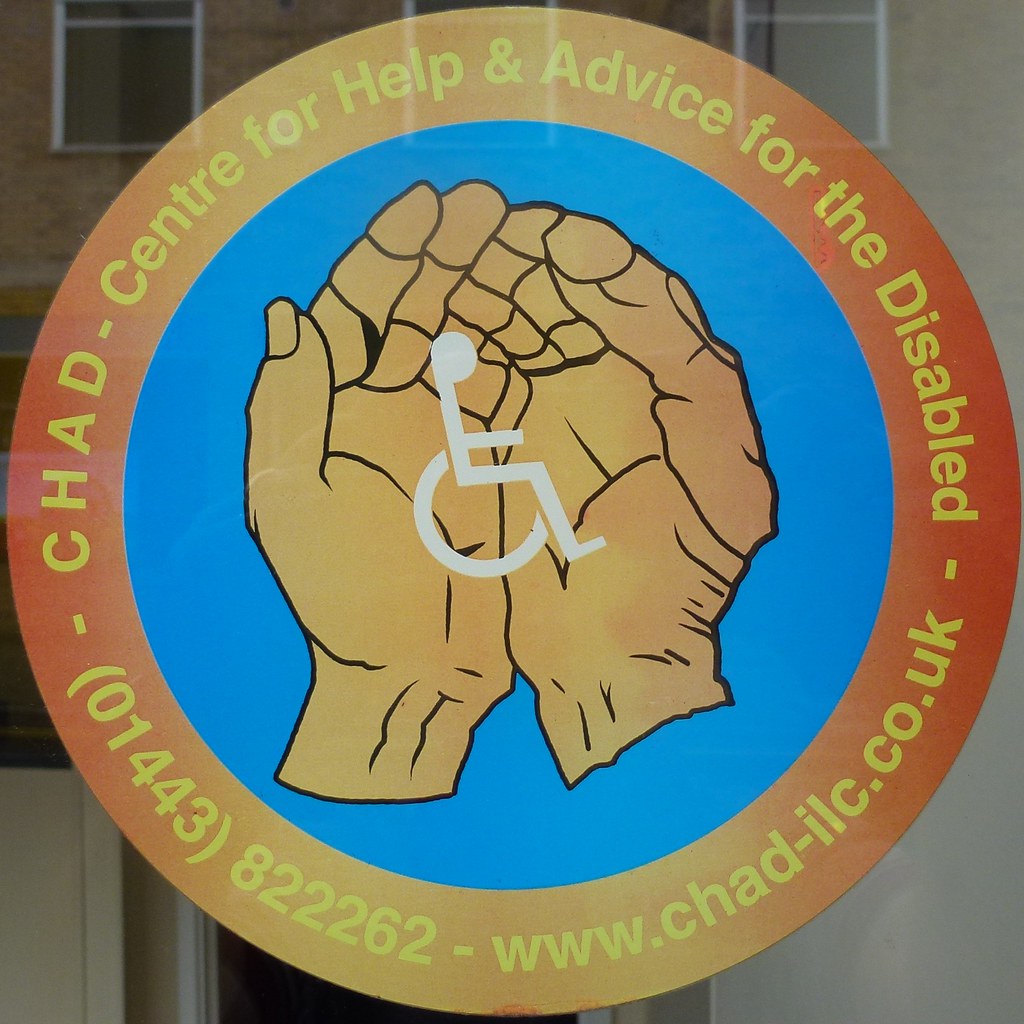This color photograph, in a square format, showcases a circular sign, possibly mounted on the facade of a beige building with visible windows at the top. The sign features a vibrant gradient of yellow and orange along its outer rim, containing yellow text that reads: "CHAD, Center for Help and Advice for the Disabled," along with the contact number "01443 822262" and the website "www.chad-ilc.co.uk." This text encircles the central theme of the sign. Inside this rim, a lighter blue circle houses a pair of flesh-toned hands, illustrated as if gently cradling something. Within these hands is the universally recognized white symbol for disability—a stick figure in a wheelchair—outlined in black. The composition of the image is representational and realistic.